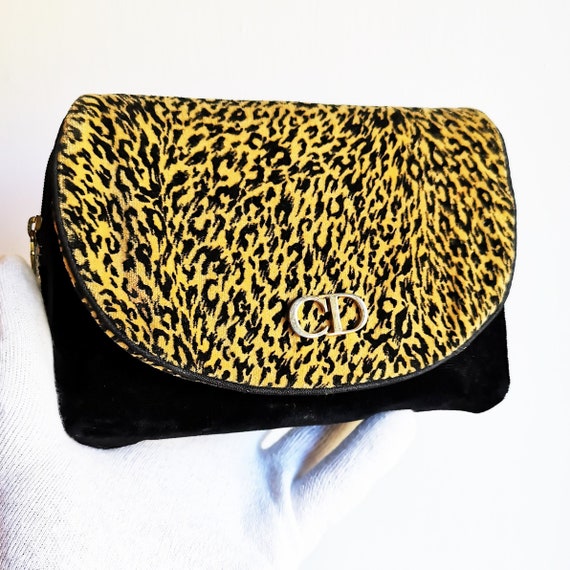This photograph showcases a stylish black handbag set against a white fabric background with noticeable folds. The focal point of the image is the rectangular black base of the handbag, which features a soft, fuzzy texture. The flap of the handbag is a striking half-moon shape adorned with a vibrant cheetah print in orangey-yellow with black curved spots, resembling a jaguar pattern. Prominently displayed at the center bottom of this flap are the gold 3D letters "CD," adding a touch of elegance. The left side of the handbag features a shiny gold zipper tag hanging down, catching the light. The white fabric backdrop is draped unevenly, with golden light filtering through in certain areas and deep gray-blue shadows accentuating the folds.